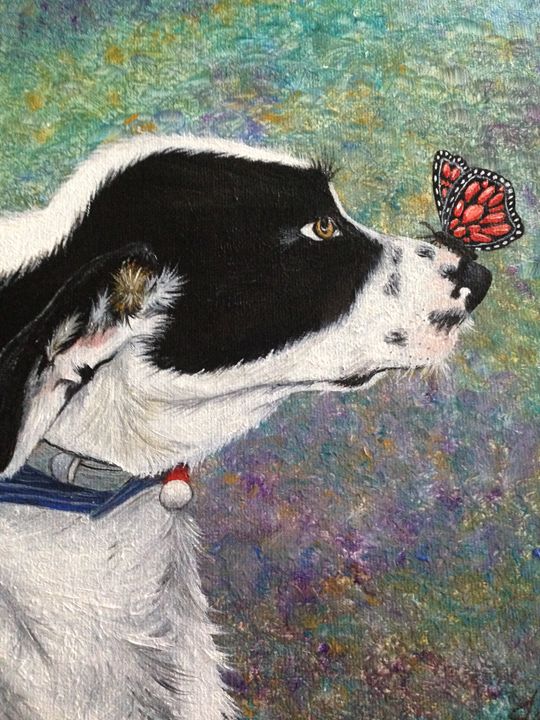This image depicts a vibrant oil painting of a black and white dog against an abstract, multi-colored background. The dog, predominantly white with a black-furred face, ears, and a few black spots on its nose, is facing towards the right. Around its neck, it sports a blue collar with a red tag. Perched delicately on the tip of the dog's nose is a butterfly with striking red and black wings. The background canvas bursts with an array of colors, including green, yellow, purple, red, blue, orange, pink, violet, and brown, possibly representing a flowered field. The combination of the dog's poised expression and the intricate details of the butterfly adds a harmonious charm to the colorful, abstract setting.